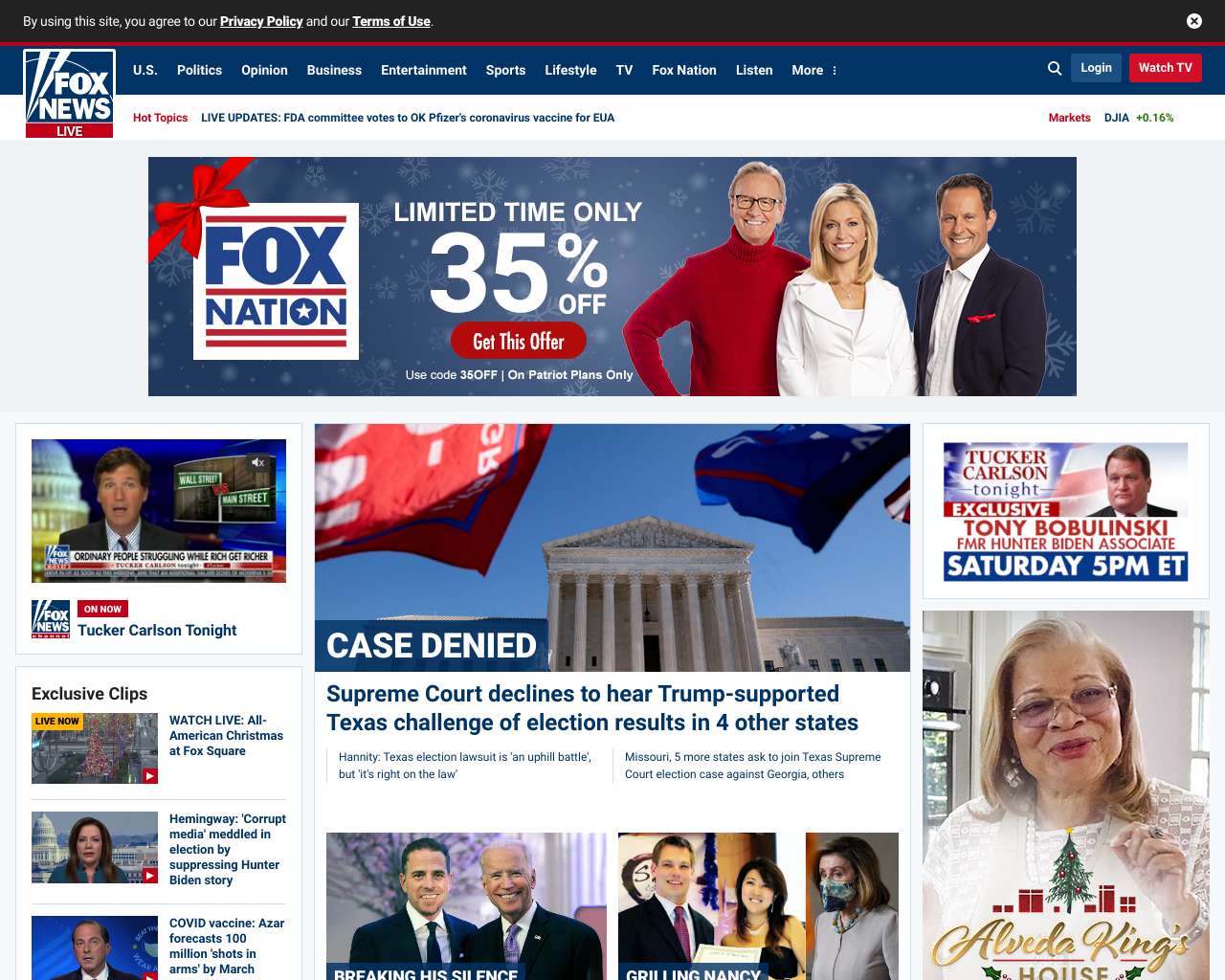This screenshot captures the Fox News homepage, prominently displaying an advertisement for Fox Nation offering a 35% discount along with a promo code. The main headline reads: "Case Denied! The Supreme Court Declines to Hear a Trump-Supported Texas Challenge of Election Results in Four Other States." 

Tucker Carlson’s segment, "Tucker Carlson Tonight," is currently on air, focusing on economic struggles. The page features exclusive clips and links to live and recorded segments, including a Christmas special and various political commentaries. Highlighted stories include the Supreme Court’s decision on the election challenge, Tony Bobulinski’s exclusive interview on "Tucker Carlson Tonight," an interview featuring Alveda King’s elaborately decorated house for Christmas, and other notable news stories.

The typical website layout includes sections for live broadcasts, breaking news, opinion pieces, and other categories. Further down the page, there are stories involving Joe and Hunter Biden, and a piece discussing Nancy Pelosi. The collection of current headlines and features represents the broad spectrum of news and opinions circulating on Fox News at the time of the screenshot.